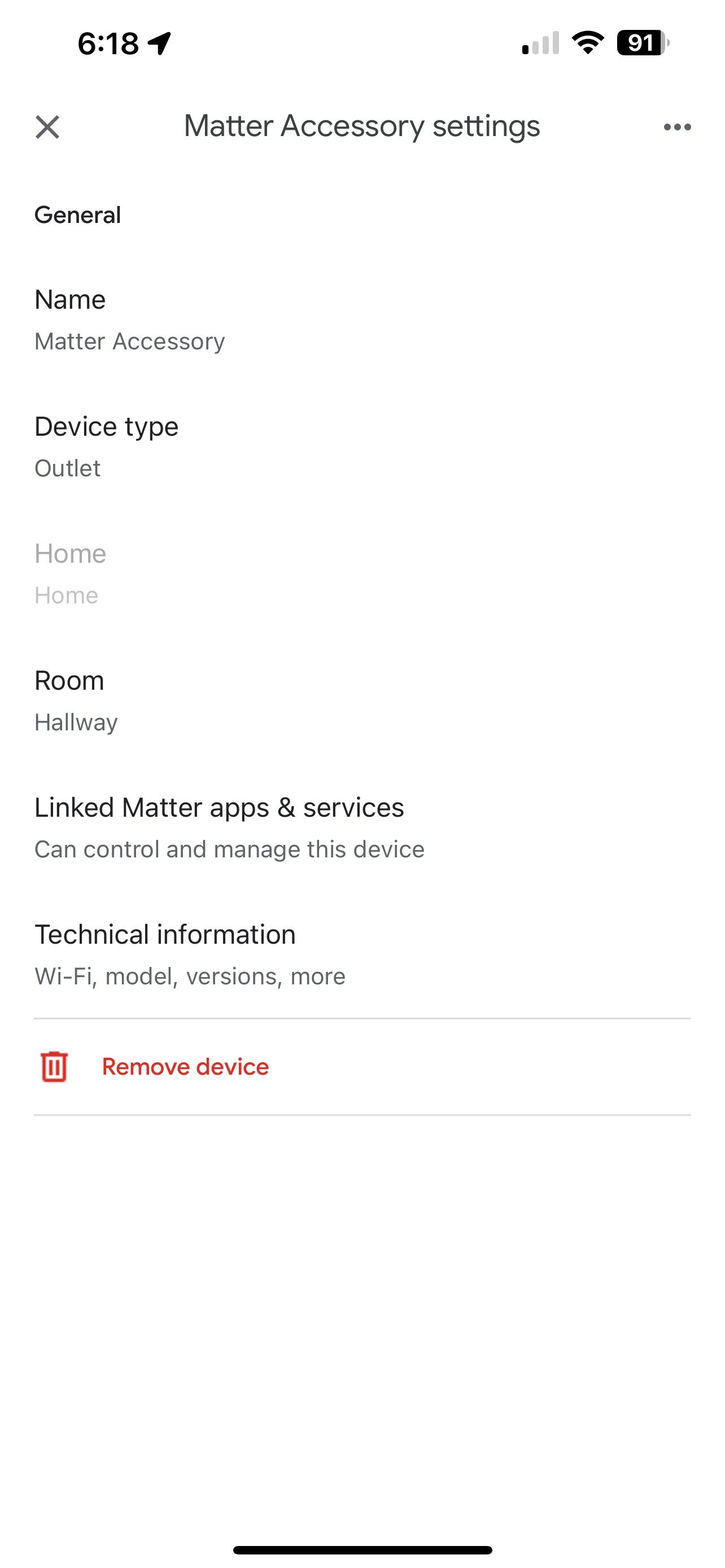This image is a screenshot taken from a cell phone, showcasing a white background. At the very top in black print, the time is displayed as 6:18, accompanied by a small airplane icon indicating airplane mode. Adjacent to this, the battery life is shown at 91%, and Wi-Fi connectivity is indicated by full signal bars.

Moving down the screen, on the left side, there is a prominent "X" icon. Next to this, there's some space followed by the text "Matter Accessory Settings" and three horizontal dots.

Further down, the section titled "General" appears. Underneath "Name," "Matter Accessory" is displayed in gray print. The next section, "Device Type," has "Outlet" written below it.

The label "Home" is displayed in gray print twice, with the second instance being more faint. 

Continuing down, the word "Room" is shown in black print. Directly below, "Hallway" is written in gray print.

The section titled "Linked Matter Apps and Services" states in gray, "Can Control and Manage this Device." Following this, the section "Technical Information" lists "Wi-Fi, Model, Versions," and the option to view "More."

At the very bottom, there is a red trash can icon with the text "Remove Device" written next to it.